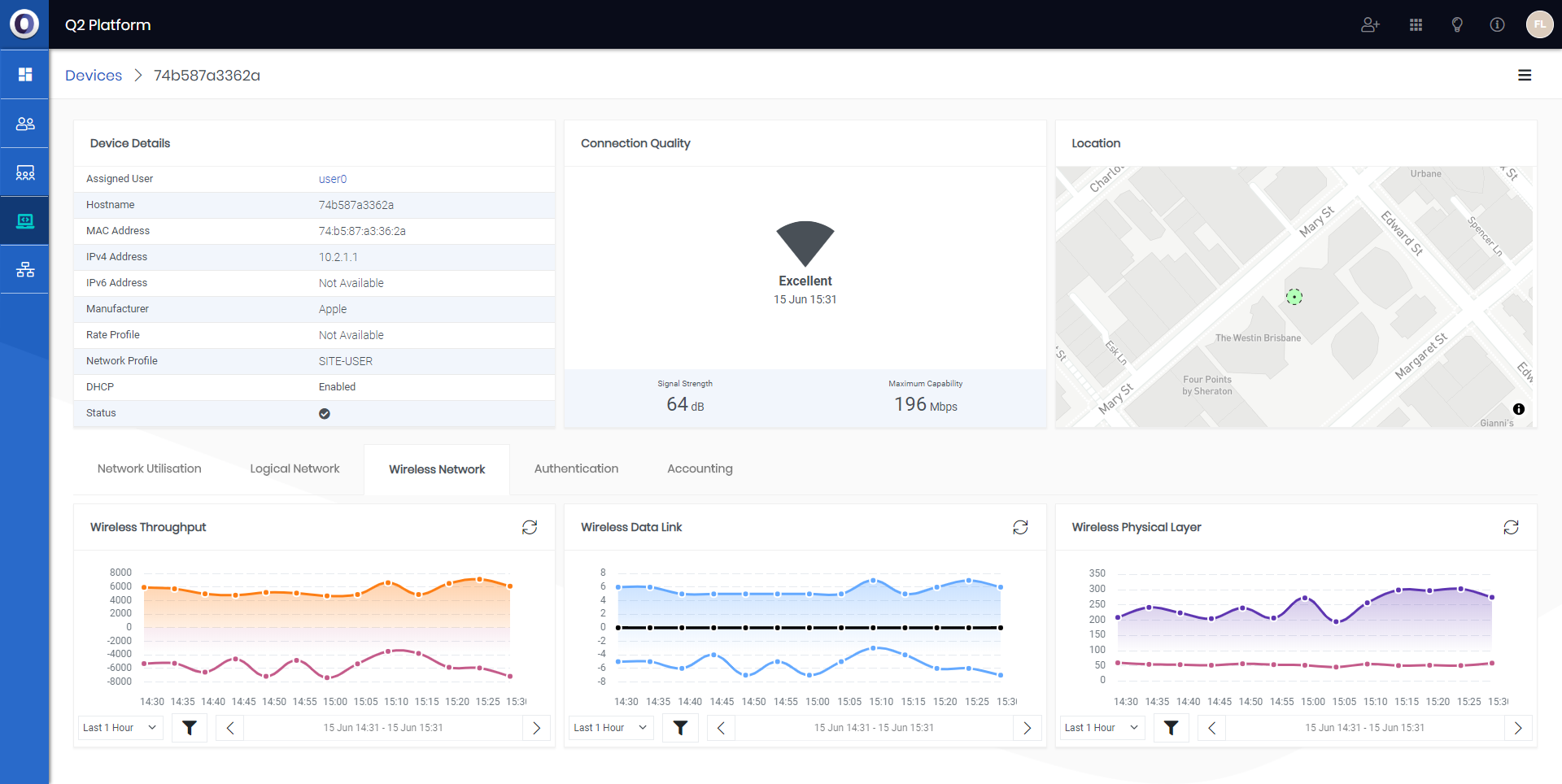The image displays the Q2 platform interface, prominently featuring a black van icon on a white background at the top left. On the right side, there is an "Add Contact" button next to a grid consisting of nine smaller boxes arranged in a 3x3 format. The interface also includes an icon of a light bulb and a circular symbol with the letters "FL."

On the left side of the image, there are four interlocking squares and an illustration of three people looking at a highlighted monitor, which reads "Devices 74B587A3362A." The details of the selected device are as follows:

- **Assigned Users**: user0
- **Host Name**: 74B (matching the device number above)
- **MAC Address**: 74B587A3362A
- **IPv4 Address**: 10.2.1.1
- **IPv6 Address**: Not available
- **Manufacturer**: Apple
- **Rate Profile**: Not available
- **Network Profile**: Site user
- **HDHCP**: Enabled
- **Status**: Checkmark (indicating it is active)

Additionally, a chart displays wireless throughput, and another graph shows wireless data link connection quality, marked as "Excellent" as of 15 June, 15:31. The signal strength is indicated at 64 dB, with a maximum capacity of 196 Mbps.